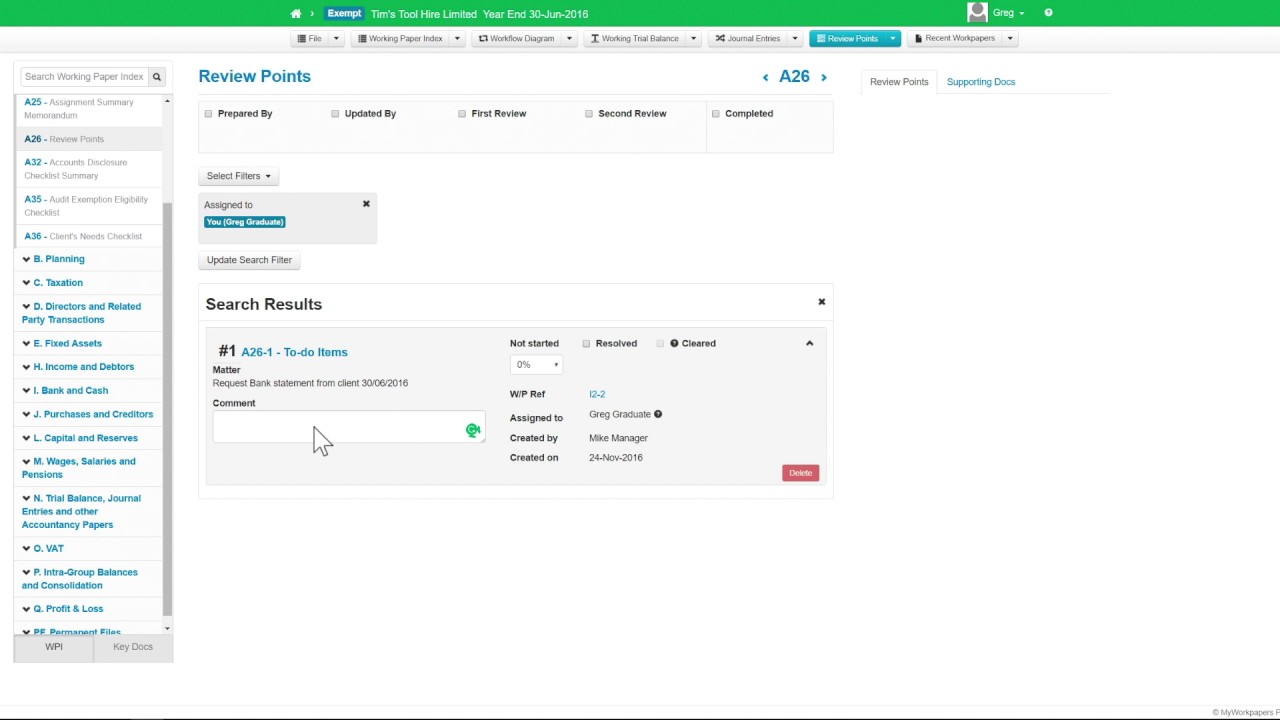In the picture, the background is primarily white. At the top, there is a green rectangular box containing white characters that resemble a small white box. Below it, a blue excerpt is visible with a white section labeled as "trial." To the right, there is a small circle and an icon of a person. 

Moving downwards, a light blue box features several headings across it, with one of them highlighted in blue. Below this section, to the left, there is a search box. Adjacent to the search box are boxes outlined in purple, with a purple slider bar on the right side. The left part of this area is heavier in purple at the top, gradually becoming lighter towards the bottom. There are also several items listed in blue print along with down arrows. One of the boxes appears to be labeled "VPN" and "key something."

On the right side, the text "review points" is displayed in blue, along with fields labeled "prepared by," "updates by," "first review," "second review," and "completed," each accompanied by a small box. Above this section, there are left and right arrows with the number 826 between them, labeled "review parts" and "shopping order."

Additionally, there are several blue boxes. The top blue box is very small, followed by a larger box labeled "assigned to," shaded in bright blue, with "you" written inside it. In the top-right corner of this area, there's a tiny X. Further down, there are up-down arrows with "update" and "select file" options, alongside "search results." The first result is highlighted in blue, showing a name and a search box with a green element and an upward-pointing arrow. To the right of this section, several smaller boxes are present and to their far right is a red button.